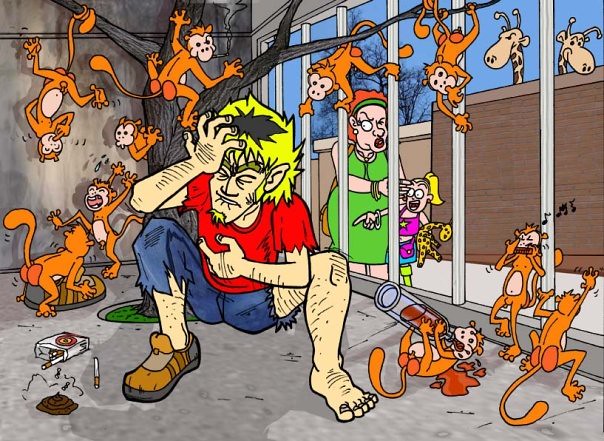The image is a detailed cartoon, drawn in a style reminiscent of MS Paint with bold black outlines and a lack of shading, giving it a comic book appearance. It depicts a chaotic zoo scenario where a disheveled man, resembling someone raised by wolves, is confined to a cage filled with lively monkeys. This man has unkempt blonde hair, a torn red shirt, ripped blue pants with one missing shoe, and he appears visibly distressed, sucking his lip with eyes closed and hand on his head. Surrounding him are about ten mischievous orange monkeys with tan bellies and faces, engaged in various antics: one plays a harmonica, another drinks what looks like alcohol, while others dance, climb a tree within the enclosure, and show off their red butts. There is also a pack of cigarettes and a pile of poop near the man. Outside the cage, to the top right, stand a woman and a child, either a mother and daughter or grandmother and granddaughter, observing the scene. In the distant background, two giraffes can be seen peering over a wall, completing the zoo environment.